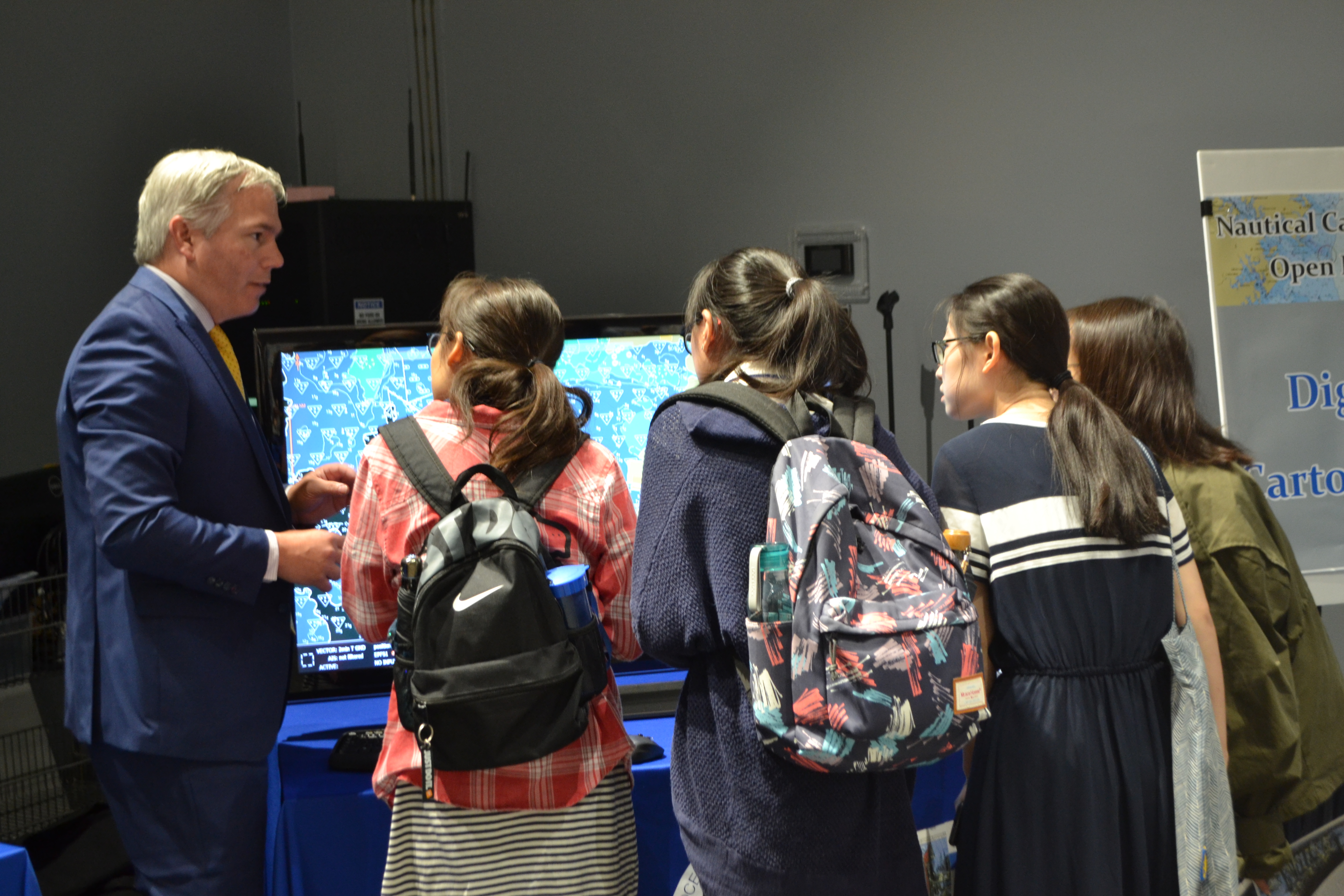In this photograph, an older gentleman, seemingly in his 50s or 60s, with gray hair and dressed in a dark blue suit paired with a yellow tie, stands to the left of the frame. Positioned before a large television monitor, approximately 50 inches in size and displaying light blue and white patterns, he appears to be either a teacher or a tour guide conducting a presentation. To his right, four young Asian women, possibly students, gather closely, listening intently to him. They all have long black hair pulled into ponytails, and two of them carry backpacks—one with a black Nike emblem and another with a dark color and floral patterns. The women are focused on the man and the screen as if learning something new, standing in an environment that might be a conference, an exhibit, or a booth. A sign next to the setup seems to read "nautical" and "DIG," indicating a possible nautical-themed exhibit.